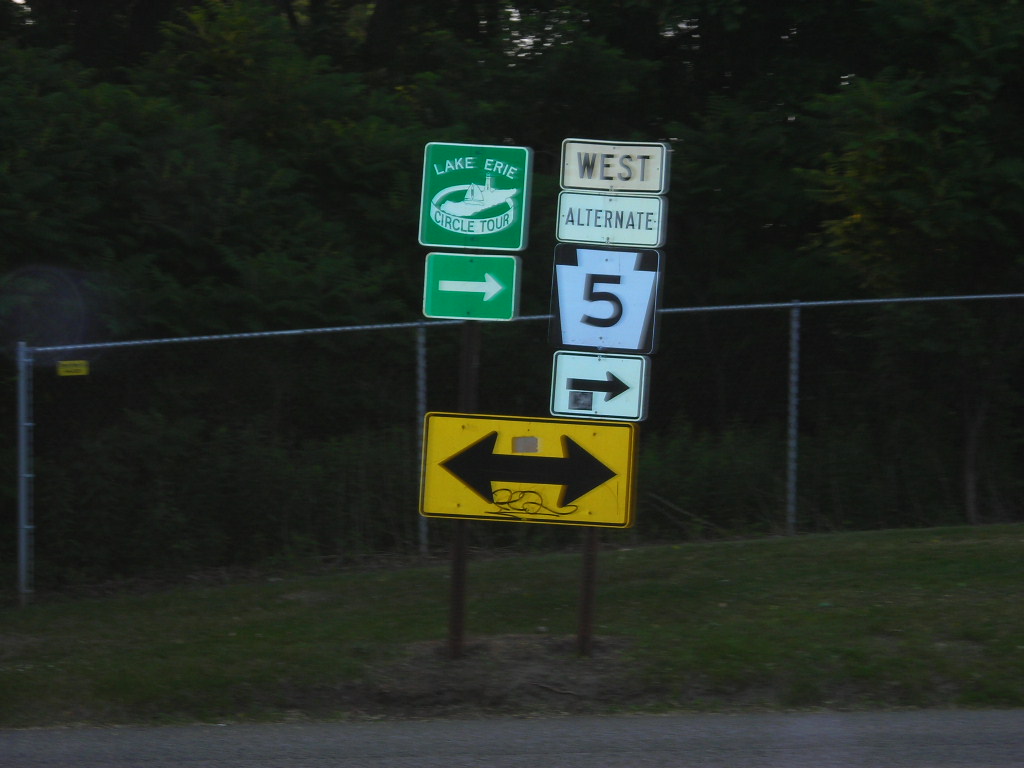This nighttime outdoor image features an arrangement of traffic and street signs mounted on two slender poles, set within a grassy area that transitions into a densely wooded background. Central to the composition is a green, square sign at the top reading "Lake Erie Circle Tour." Beneath this is a rectangular sign with an arrow pointing to the right, and another sign saying "West Alternate 5" in various shapes and colors, including a white arrow directing westward. A smaller, rectangular yellow sign with black arrows pointing both west and east is positioned at the bottom, flanked by some graffiti. The signpost is surrounded by a patch of grass enclosed by a chain-link fence, topped with a pole and situated in a darker, lush woodland area. The scene is subtly lit, hinting at early evening or night, with just enough light to distinguish the intricate details of the signs and the dense greenery in the background.